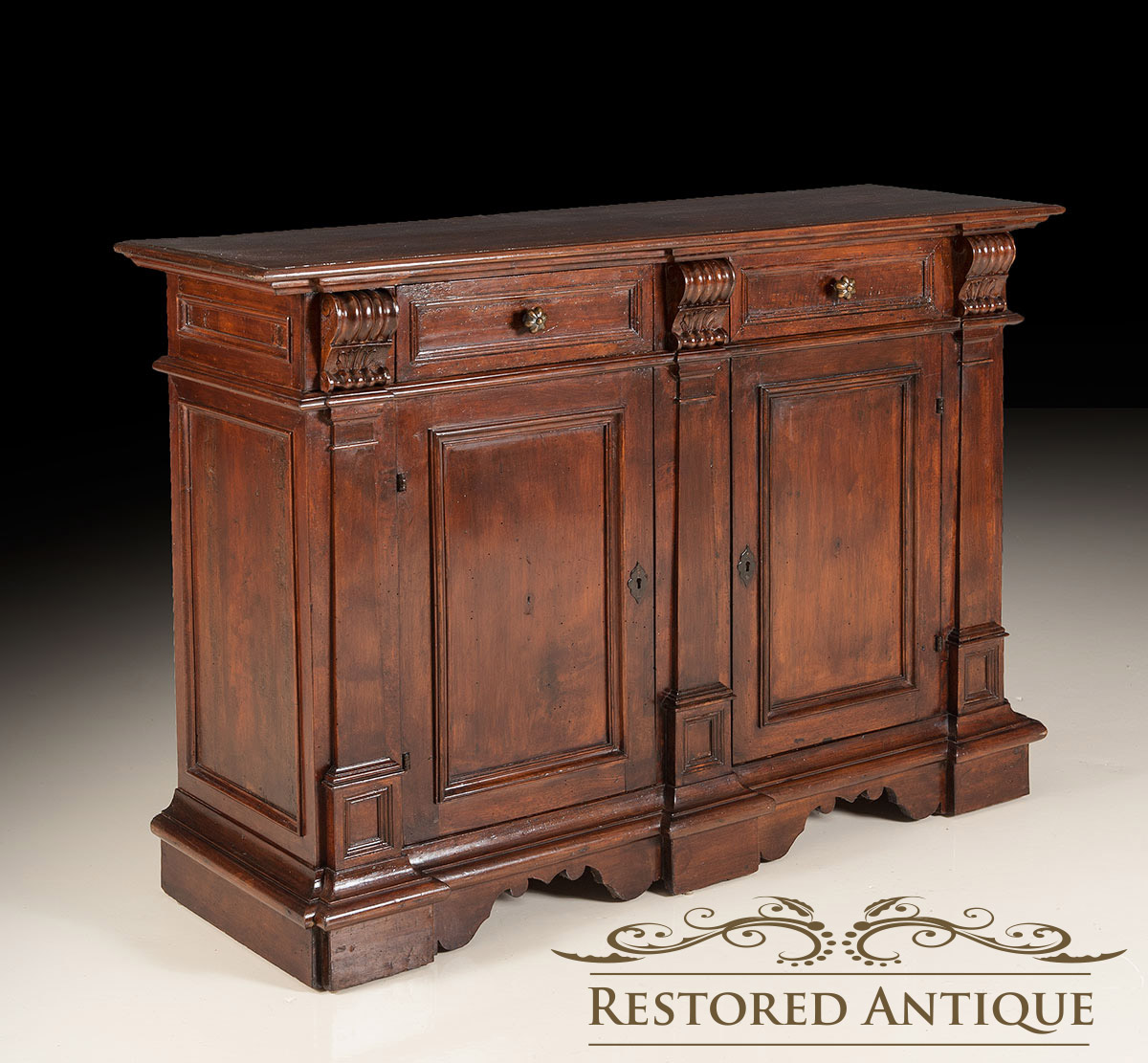The image features a vintage wooden cabinet with a distinctly old design, showcasing a blend of brown and red paint. The cabinet consists of four compartments: two pull-out drawers positioned at the top and two doors leading to larger shelves at the bottom. The handles of the drawers are clearly visible, as well as keyholes centered on the bottom doors, emphasizing its antique character. The background of the photograph transitions from black at the top to white at the bottom. A logo in the bottom right corner reads "Restored Antique," indicating the cabinet’s refurbished nature.